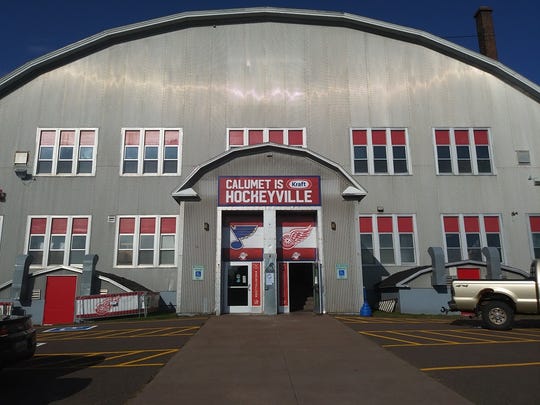The image features a prominent silver, metal building with a distinctive semi-circular, dome-shaped roof under a clear, blue sky. The building appears to be at least two stories high, as evident from the numerous windows framing the structure - sets of three windows on the upper level, and sets of four on the lower level, with a partial view of a fifth window. Each window is adorned with red accents and framed in white. Prominently, the words "Calumet is Hockeyville" are displayed in white lettering on a red background above the central doorway, accompanied by a probable Kraft logo above, although it's partially obscured. Additionally, logos for the St. Louis Blues and Detroit Red Wings can be seen above each of the two main doors. The front of the building is accessible via a pathway that cuts through a blacktop parking lot marked with yellow lines, featuring a visible gold truck and a black car parked in view. The right side of the building is also marked by a brick chimney, accenting the overall structure. This detailed scene likely depicts a community hockey arena, as suggested by the signage and overall layout.